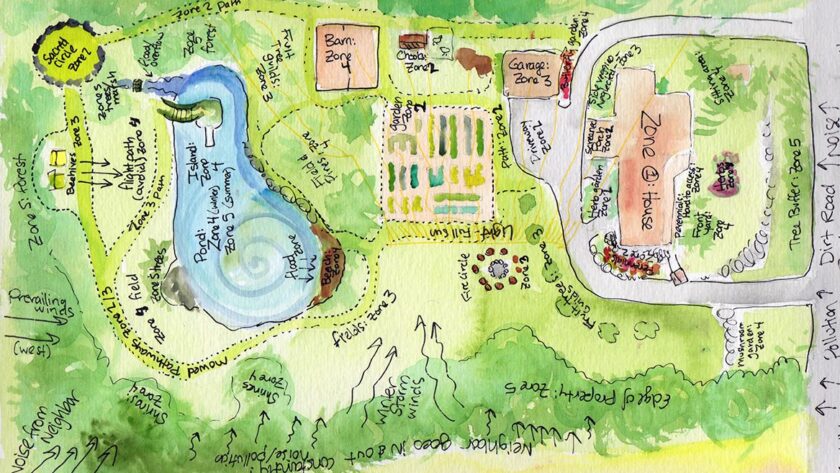This detailed watercolor map vividly illustrates a property with various zones and features. The map uses an array of colors, including blue, light blue, dark blue, light green, medium green, and dark green, to differentiate between areas and elements. Labeled zones include Barn Zone 4, Garage Zone 3, and House Zone 1, each section clearly demarcated with black pen labels. A prominent body of water, illustrated in shades of blue, occupies a substantial portion of the map. Surrounding this are green areas representing lush foliage and grassy fields, adding to the verdant appearance of the scene.

Arrows on the left side of the map, marked with "Prevailing Winds," provide directional context, most likely indicating seasonal wind patterns relevant to the property layout. Various illustrations such as a flower bed and a garden enrich the depiction, suggesting an organized and well-maintained outdoor space. The map also includes roads and pathways, further detailing the property’s navigation routes.

From the density of text labels to the meticulous drawing style, this map seems both informative and decorative. It may serve to demarcate different functional areas and features of a property. The presence of a "big hedge" or potential tree line at the property's edge hints at a clear boundary separating it from neighboring areas, ensuring privacy and defining space usage effectively. Overall, this map offers a childlike charm yet maintains a sophisticated level of architectural detail.